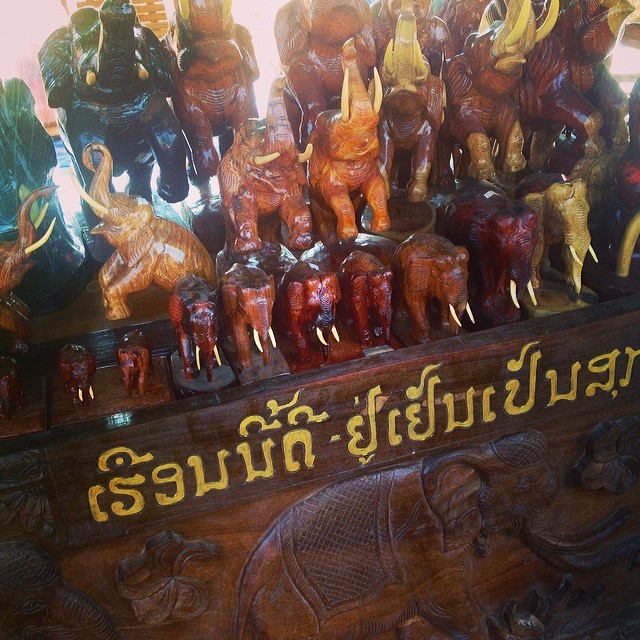This photograph captures a stunning display of intricately carved elephant statues arranged on a dark wooden chest, which is elegantly adorned with a carved large elephant in low relief and gold lettering that appears to be in either Thai or Hindi. The chest showcases a wide array of elephant carvings, comprising around 15 to 20 statues of varying sizes and intricate designs. The elephants, crafted from a variety of materials that seem to include both wood and stone, exhibit a spectrum of colors ranging from pale yellow and golden hues to dark reddish browns and black. The smallest elephants, possibly representing baby elephants, are positioned on the bottom shelf, some of which lack tusks. The middle shelf features slightly larger elephants, and the top shelf displays the largest ones, including a notably prominent black elephant on the top left. These sculptures, some standing on all fours and others rearing on their hind legs, beautifully capture the cultural essence and artisanship, likely drawing inspiration from Indian or Thai artistry. The overall scene, filled with warm earthy tones of browns, oranges, and reds, is complemented by the meticulous carvings of elephants and floral patterns, reflecting a rich cultural heritage.